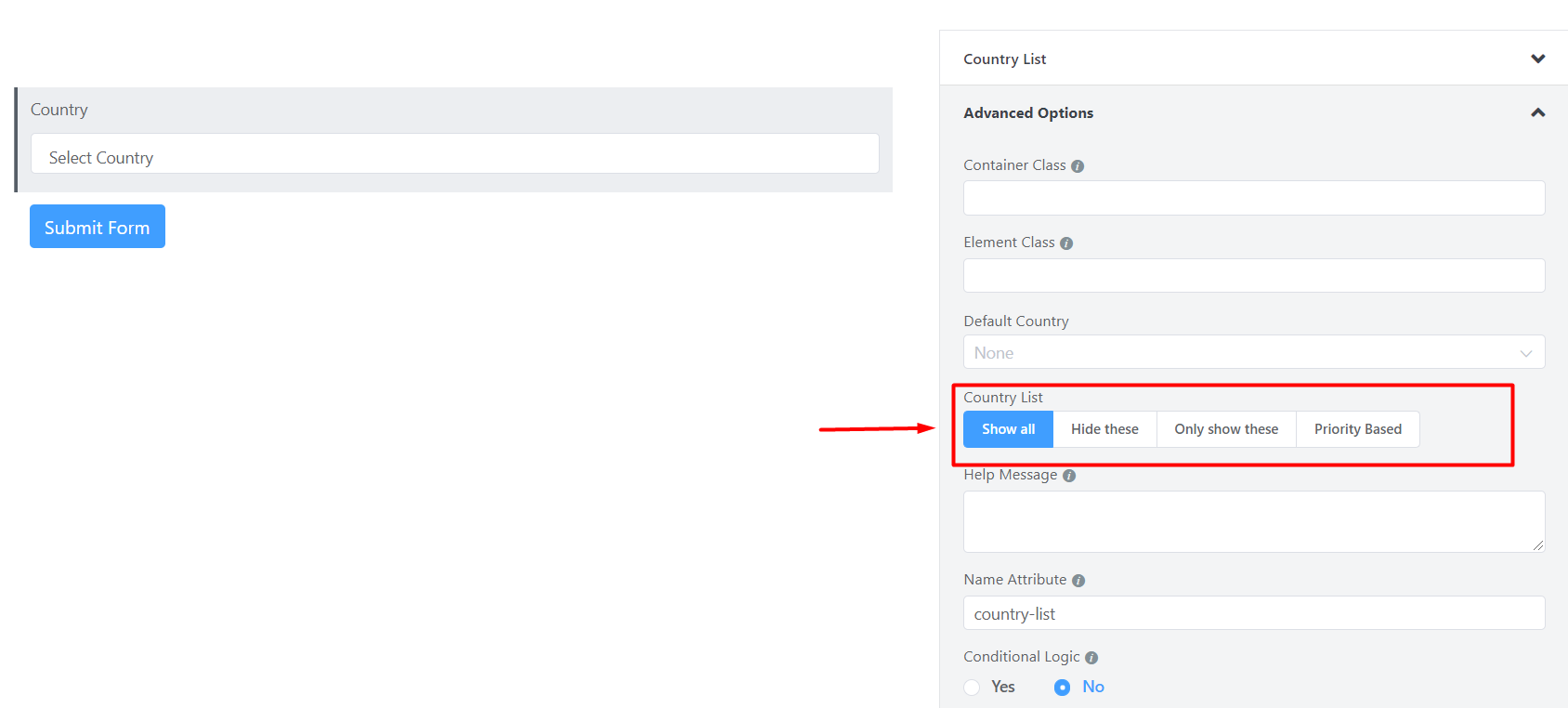The image showcases a form interface divided into two main sections against a white background, with a focus on country-related input fields.

**Left Side:**
- There are text fields labeled "Select Country" for the user to input options.
- A prominent blue button with white text labeled "Submit Form" is displayed.

**Right Side:**
- The section is headlined with "Country List."
- An "Advanced Options" button is available.
- Below it are several fields: "Container Class," "Element Class," and "Default Country," followed by a list of countries.
- A "Show All" button is highlighted, surrounded by a red outline with a red arrow pointing towards it, indicating its importance and suggesting the user should click it.
- Additional fields include a "Help Message" text area, "Name Attribute for Country List," and a "Conditional Logic" section with Yes/No options, where "No" is currently selected.
- The input fields have a gray background, while the text fields are white, contributing to the page's straightforward and user-friendly design focused on various country-related settings and options.